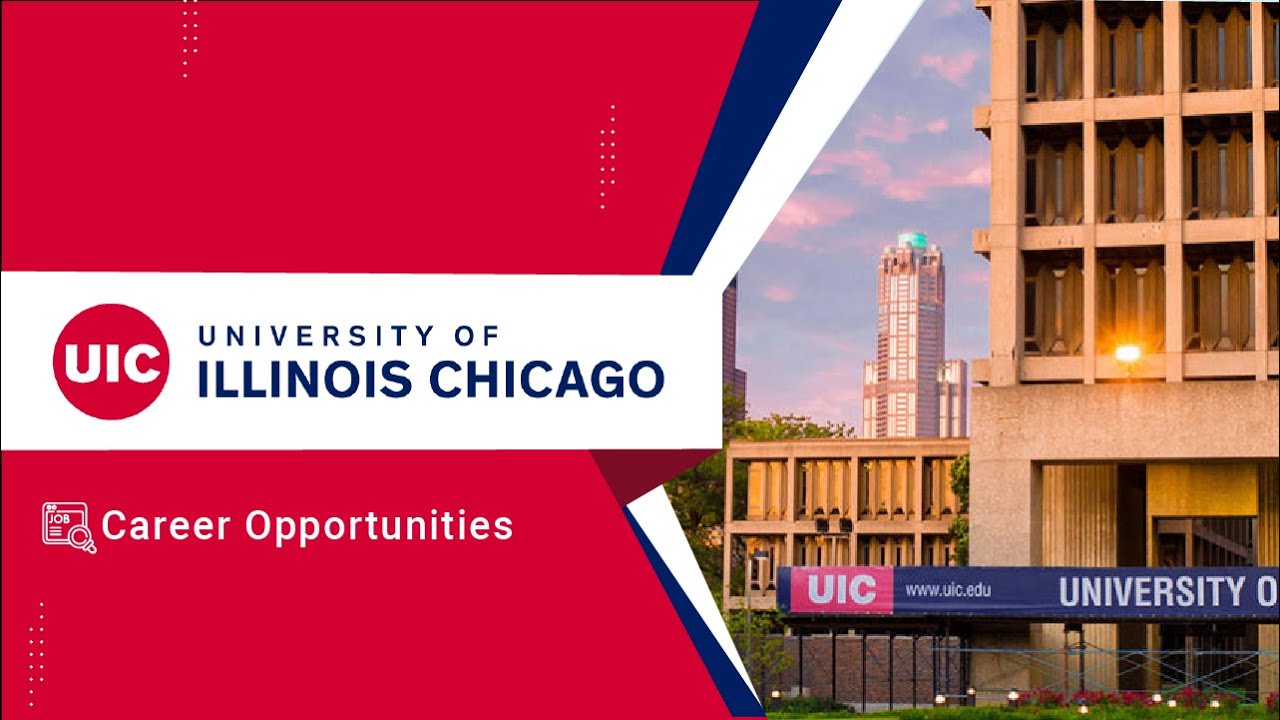The image is a visually engaging advertisement for the University of Illinois at Chicago displayed on a computer screen. Dominating the center is a large white rectangle, prominently featuring a red circle with the initials "UIC" in bold, white, capital letters. The left side of the screen is primarily filled with a vibrant red background, accentuated by two vertical lines of decorative dots. 

Towards the bottom of the screen, an appealing cartoonish icon of a microphone is accompanied by the text "Career Opportunities" in white. Moving to the left side, the screen features a diagonal strip pattern with navy blue transitioning into white, adding a dynamic visual element.

On the right side of the screen, the background showcases large, modern buildings, one of which has a teal accent at the top and seems to reflect the setting sun on its windows. The partial text "UIC" and "University O" further hints at the promotional content, although it is cut off in this view, adding a sense of intrigue.